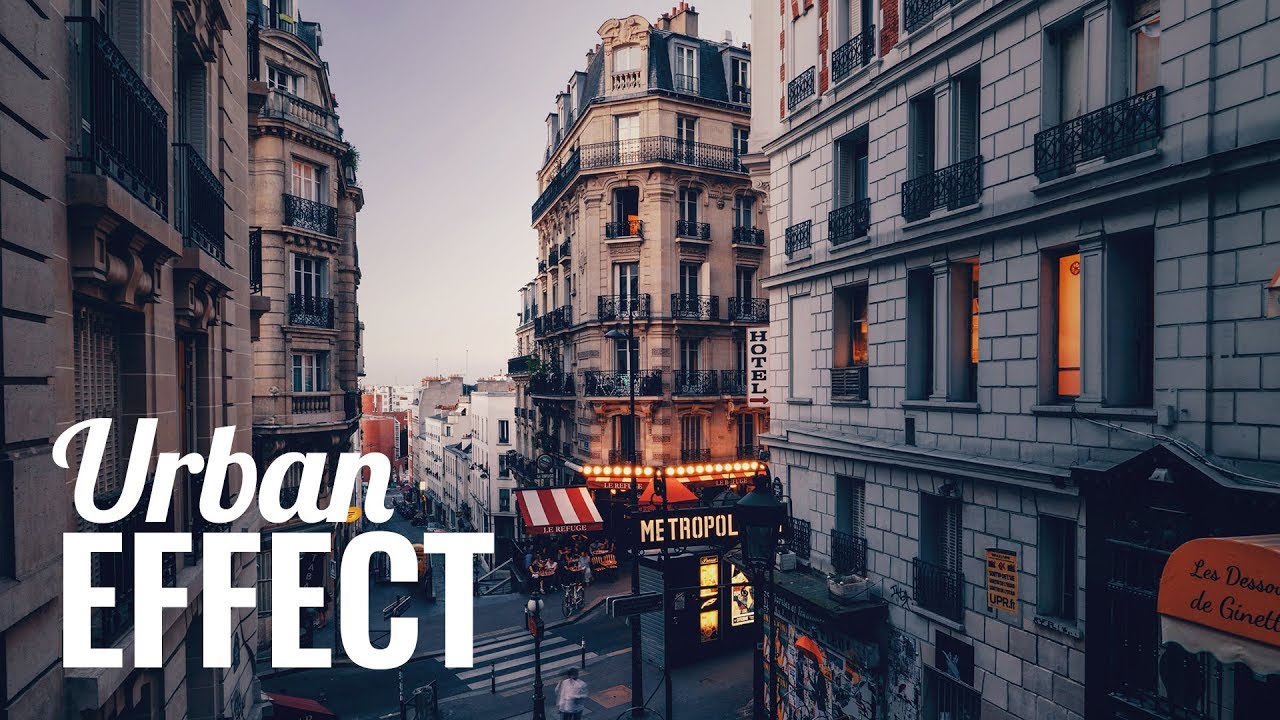The image is a highly detailed, photorealistic advertisement featuring an urban scene, likely from a French or Swiss city. Dominating the left-hand side are two large beige buildings, with a distinct light gray building and another beige structure on the right. All buildings appear to be made of brick or pale sandstone, showcasing their intricate patterns. In the middle of the scene is a busy street, filled with people walking, some on bicycles, and cars. The street is characterized by its compact and bustling nature, resembling a shopping or downtown district. The buildings on the street display various commercial signs, including a notable hotel sign with a red arrow and a blue-striped awning labeled "Metropole." Additional signage includes a message about a last day event and text in a different language, suggesting international appeal. At the bottom left corner of the image, the phrase "Urban Effect" is prominently written in large white letters, adding to the sophisticated urban theme of the advertisement.